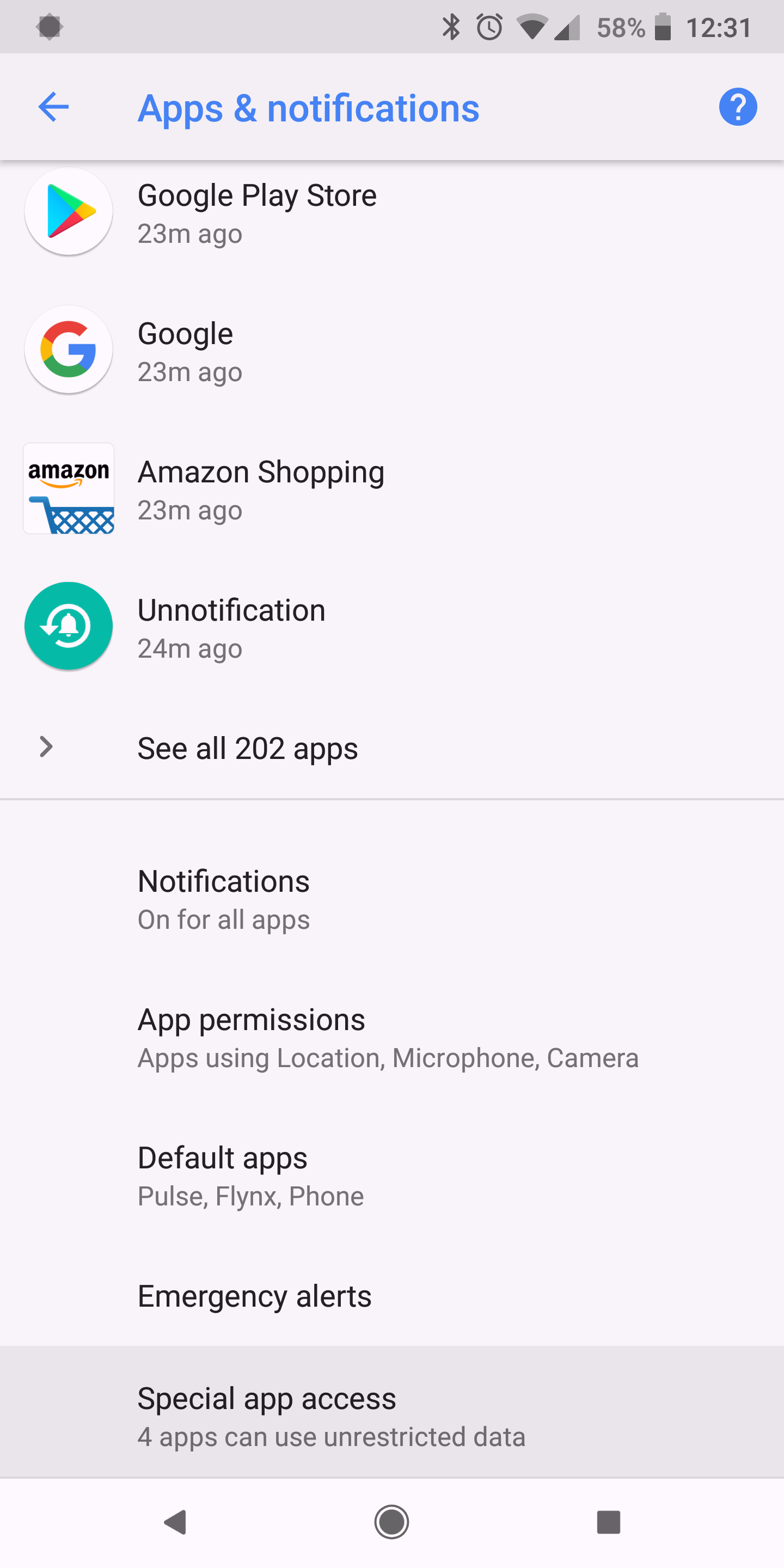This image is a detailed screenshot of a cell phone's screen, showing the "Apps and Notifications" section. The image clearly indicates that it is a cell phone screen due to the standard icons in the upper-right corner: a battery icon showing a 58% charge, a time display, a signal strength indicator, and an alarm clock icon. This area is highlighted within a gray rectangle stretching across the screen's width.

Beneath this is a thinner, lighter gray rectangle featuring a back arrow on the left, followed by the title "Apps and Notifications" in blue text and a help icon—a blue circle with a white question mark—in the right corner.

The main content reveals a list of the device's applications and their recent activity. The first item is the Google Play Store, accessed 23 minutes ago, accompanied by its distinctive logo in a white circle. Below it, the "Google" app is listed similarly. Further down, the list includes other frequently used apps like Amazon Shopping, as well as a notification that there are a total of 202 apps installed on the phone, with an option to view them all.